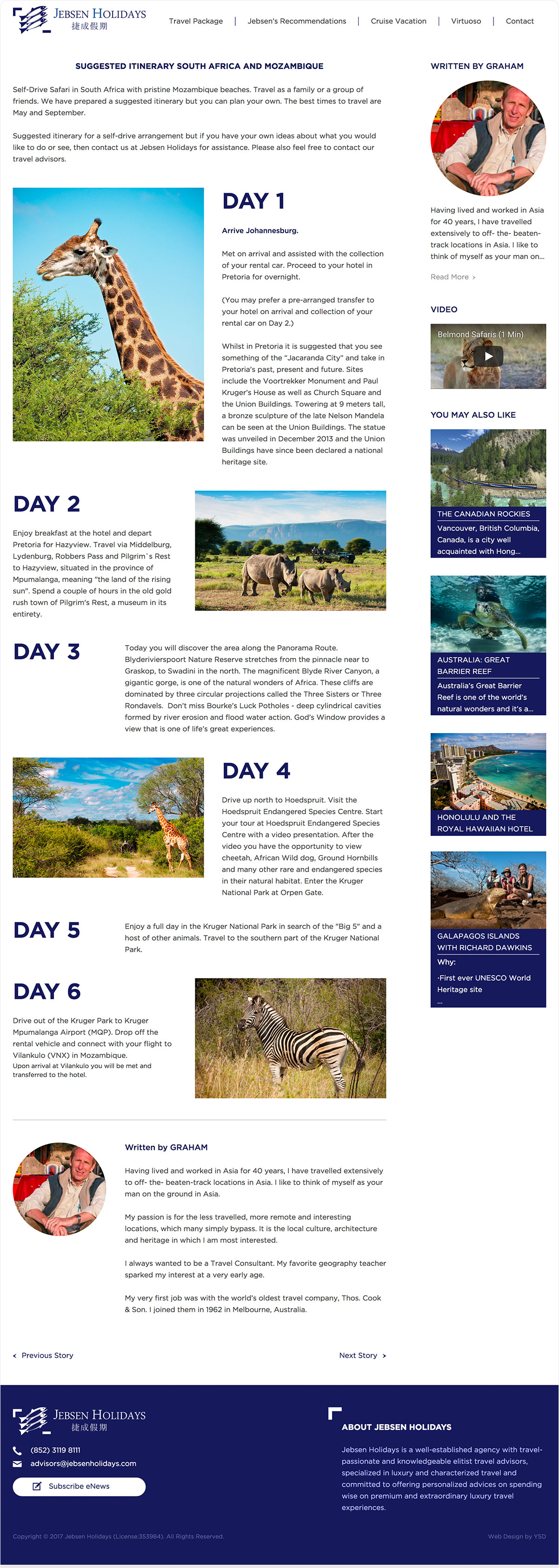Here is a detailed and cleaned-up caption for the image described:

---

The image is a vertical, rectangular screenshot, appearing to be taken from either a cell phone or a computer screen. It features a white background with black text interspersed with various animal photos. At the top left corner, the header reads "Jebson Holidays Travel Packages," followed by "Suggested Itinerary: South Africa and Mozambique."

The itinerary breakdown includes:

- **Day 1: Arrive in Johannesburg** - Accompanied by a lengthy paragraph of text, and to the left, there's an image of a giraffe standing against a backdrop of trees and a blue sky.
- **Day 2** - Detailed in another paragraph of text. To the right, there is a picture of rhinoceroses walking through the plains with a clear, blue sky above them.
- **Day 3** and **Day 4** - Each day's activities are described in their respective paragraphs. Left of "Day 4" is another giraffe image, with trees and a blue sky in the background.
- **Day 5** and **Day 6** - Continuing with textual details, adjacent to "Day 6" is a picture of a giraffe in a grassland setting.

In the screenshot's upper right corner, there is a circular photo of a smiling white man under the caption "Written by Graham." Below his picture are additional boxes featuring images and descriptions of travel destinations:
- A clickable video showing an image of a lion.
- Four travel content boxes with labels:
  - "The Canadian Rockies"
  - "Australia's Great Barrier Reef," showcasing a sea turtle in the water.
  - "Honolulu and the Royal Hawaiian Motel"
  - "Galapagos Islands"

Each box likely represents another travel package or destination available for viewing.